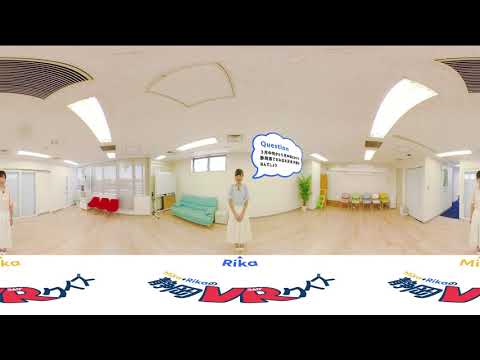The image depicts a well-lit, modern living room or possibly a lobby, characterized by its clean, angular design. The floor appears to be made of light beige, likely birch wood. The ceiling and the surrounding walls are white, and there are windows at the top of the back wall allowing natural light to flood the room. 

Centrally positioned is a young woman named Rika, dressed in a blue top and white skirt. She stands upright with her hands clasped in front of her, and there is a speech bubble emerging from her mouth, although the text inside it is too small to read and in a foreign language, presumably Japanese. On the floor below her, the name "Rika" is written alongside Asian characters and large "V-R" letters in red.

To Rika's left and right, there are cut-off images of two other women, dressed similarly in white outfits. On the far left, an additional female figure with dark hair is partly visible, with the letters "MI" below her. On the far right, another partial figure is present, with the letters "KA" underneath her.

Additional furnishings include a seafoam blue couch and three red chairs situated to the left of Rika, along with some windows behind them. To the right of Rika, there is a white wall and a green plant, accompanied by more chairs lined up against the wall. The image captures a spacious, bright environment with a mix of natural and artificial light, evoking a clean, modern aesthetic.